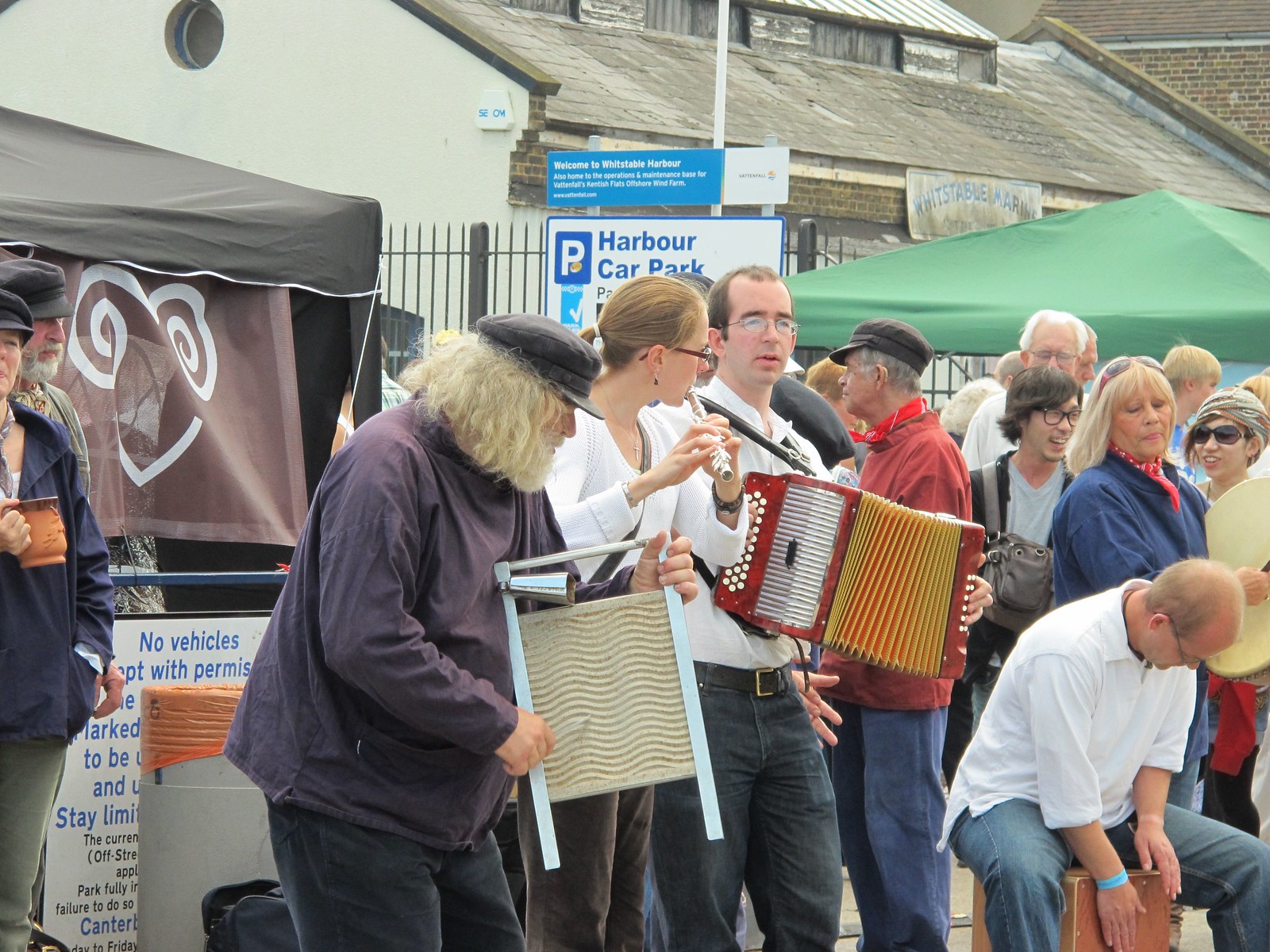In this detailed and bustling scene, we are immersed in what seems to be an outdoor festival or fair. At the heart of the image is a lively group of musicians performing energetically. Centrally located, we see an older man with gray hair, a beard, and a dark hat, donned in a black long-sleeved shirt and black pants, playing a washboard that intriguingly includes a bell. To his left (our right) stands a young woman with her hair pulled back into a ponytail, wearing a white shirt and brown pants, skillfully playing a flute while scanning the crowd. Next to her is another young man, clean-shaven with receding hair and glasses, clad in a white shirt, black belt, and blue jeans, enthusiastically playing a red accordion. Further to the right, anchoring the rhythm section on a box drum, sits an older, balding man with glasses, concentrating intently on his percussion.

The backdrop reveals a white sign partially obscured, instructing "No Vehicles Permitted," positioned by a trash can. Above, a more prominent sign reads "Harbor Car Park." On the left side, a booth—marked by a vague brown image—is part of the scene and there’s a person holding a mug nearby. The setting is vibrant with about 10 to 20 people milling around, seemingly indifferent to the musicians, hinting at the casual mingling typical of an outdoor event. In the top right, there's a green tent, adding to the festival atmosphere. This snapshot not only captures the musicians in motion but also the dynamic and informal hustle of an outdoor gathering under the daylight.